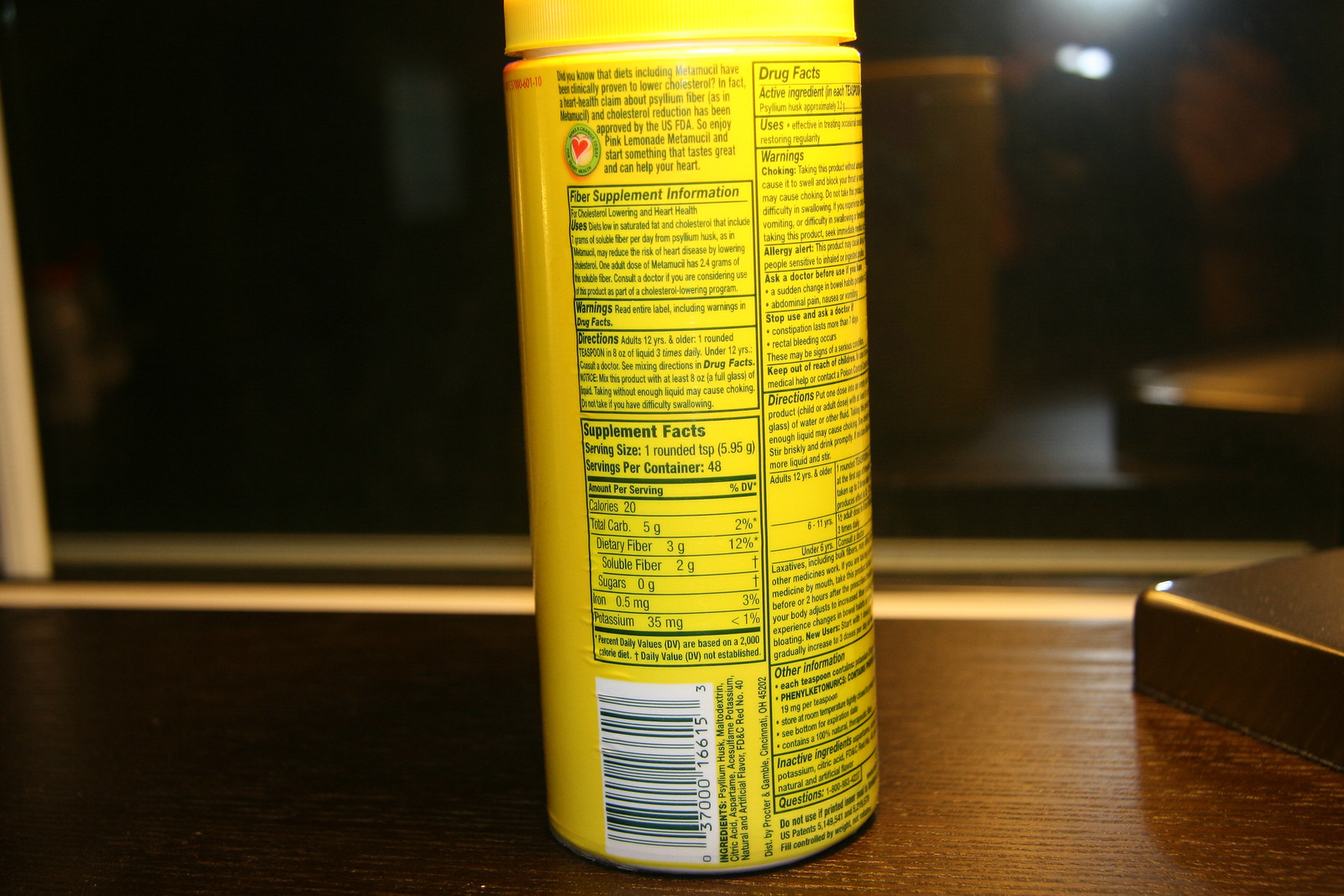The image features the back of a tall, cylindrical aluminum can with a yellow exterior. Prominently displayed on the can is a label indicating "Supplement Facts." The can is positioned on a dark wooden surface, possibly a desk. In the background, to the right of the can, a partial view of a window is visible. The window is bordered by a wood-like block with a thin, bronze frame, adding an element of sophistication to the scene. The overall lighting subtly highlights the metallic sheen of the can while casting gentle shadows on the wooden surface, creating a warm and inviting atmosphere.